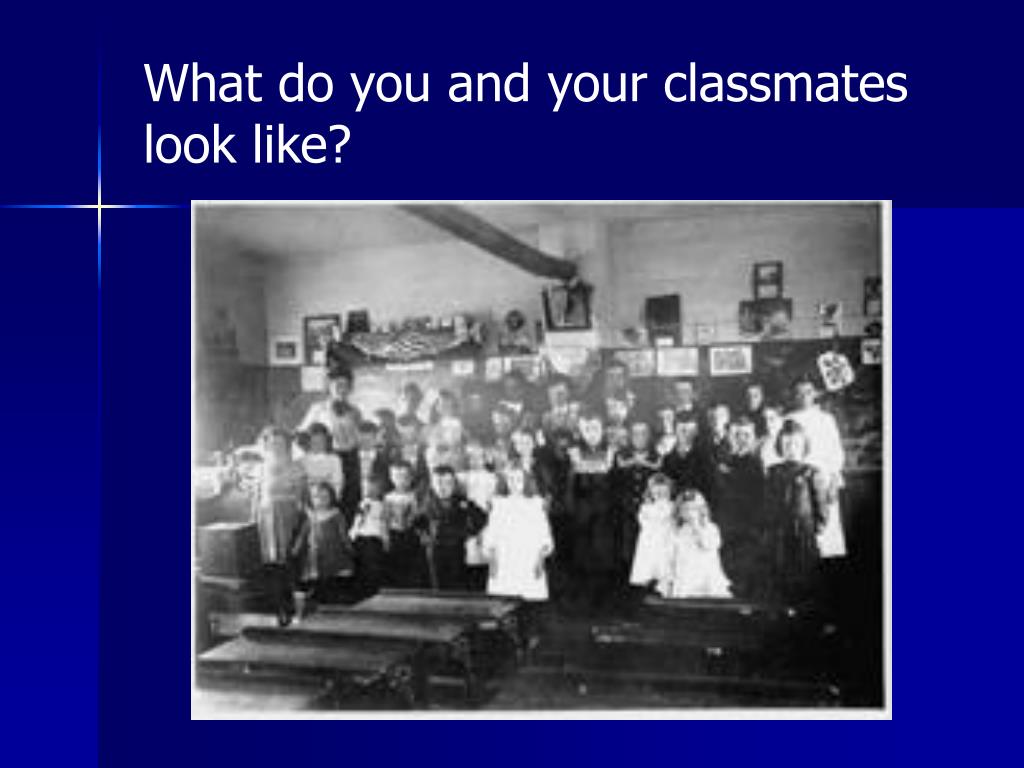The slide features a cobalt blue background adorned with geometric square designs in varying shades of blue. Prominently in the upper left corner is a white cross-shaped star that transitions into lighter blue and dark blue towards each of its four sides. At the top of the slide, in white font, is a question split into two rows: “What do you and your classmates look like?” Below this text, central to the slide, is a vertically-oriented, black-and-white photograph of an old-fashioned classroom. 

The photograph captures a class picture from the early to mid-20th century, possibly the 1920s to 1940s. It shows young school children, aged around six to ten years old, dressed in period-specific clothing, with the girls in long dresses typical of the era. The children are organized in four neat rows, and behind them is a chalkboard surrounded by various other pictures. To the back left of the classroom stands a teacher, also clad in a long dress, suggesting historical context. The classroom features wooden desks and walls, possibly with some brickwork above the wood, completing the setting of this nostalgic scene.